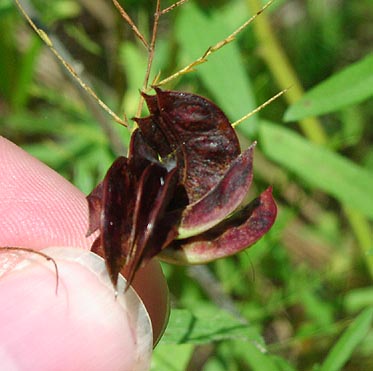The image is a very close-up, square photograph featuring a cluster of dried, purple to dark brown petals or seed pods. These are being delicately held between a person's thumb and index finger, clearly revealing the person’s trimmed thumbnail. The petals are about the size of a thumbnail and display a characteristic curved or partial U-shape, pointing in various directions. In the background, blurred green leaves and possible grass stems create a natural setting, while a tall, thin stem with grass-like seeds rises directly behind the main cluster. The scene captures the intricate details of these dried botanical elements against a vibrant, leafy backdrop.